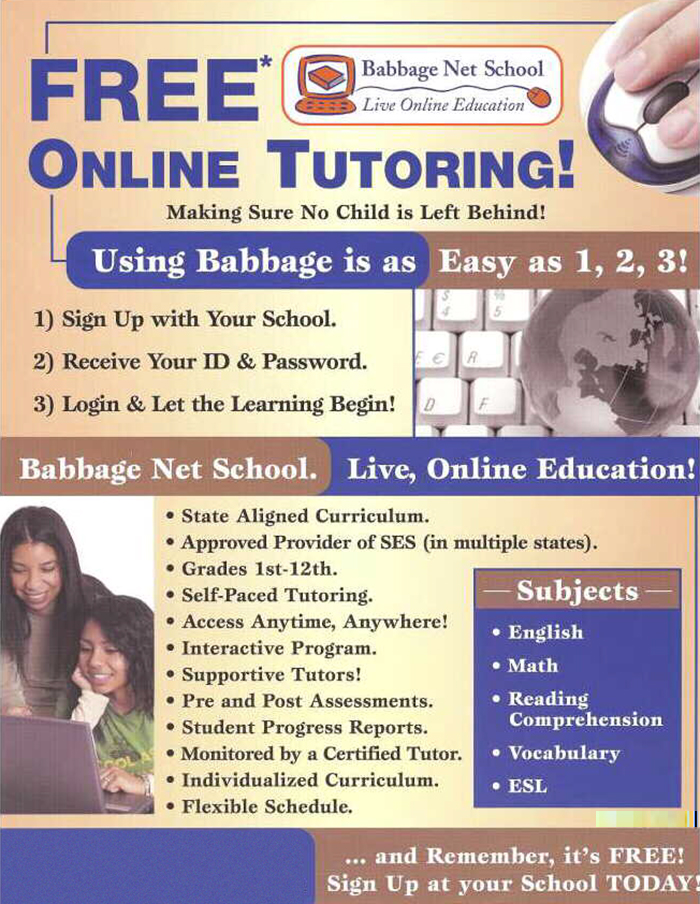**Image Caption: Comprehensive Advertisement for Babbage Net School's Free Online Tutoring Services**

The image prominently advertises Babbage Net School's free online tutoring, designed to ensure that no child is left behind. In the top left corner, large blue text boldly states: "Free Online Tutoring - Making sure no child is left behind." 

Central to the design is an engaging visual featuring a computer screen displaying an open book, symbolizing digital learning. Adjacent to this, on the right, is an image of a hand resting on a computer mouse, underscored with the text: "It's as easy as 1, 2, 3." This text breaks down the simple steps: 
1. Sign up with your school.
2. Receive your ID and password.
3. Log in and let the learning begin.

Further enriching the digital theme, an image of a keyboard with a globe overlays the right side, accompanied by the text: "Babbage Net School - Live Online Education."

Below, on the left, a photo captures a woman and a young girl keenly engaged with a laptop, emphasizing the helpful support of a tutor. This section highlights the curriculum's quality and flexibility with captions reading: "Early Aligned Curriculum," "Approved provider of SES in multiple states," and "Grades 1-12." The features listed include:
- Access anytime, anywhere.
- Interactive program.
- Supportive tutors.
- Pre and post assessments.
- Student progress reports.
- Monitored by a certified tutor.
- Individualized curriculum.
- Flexible schedule.

To the right, a list of subjects offered is prominently displayed: "Subjects: English, Math, Reading Comprehension, Vocabulary, ESL."

In the bottom right corner, a friendly reminder states: "And remember, it's free. Sign up at your school today." A simple blue border decorates the lower left of the page, adding to the overall polished look of the advertisement.